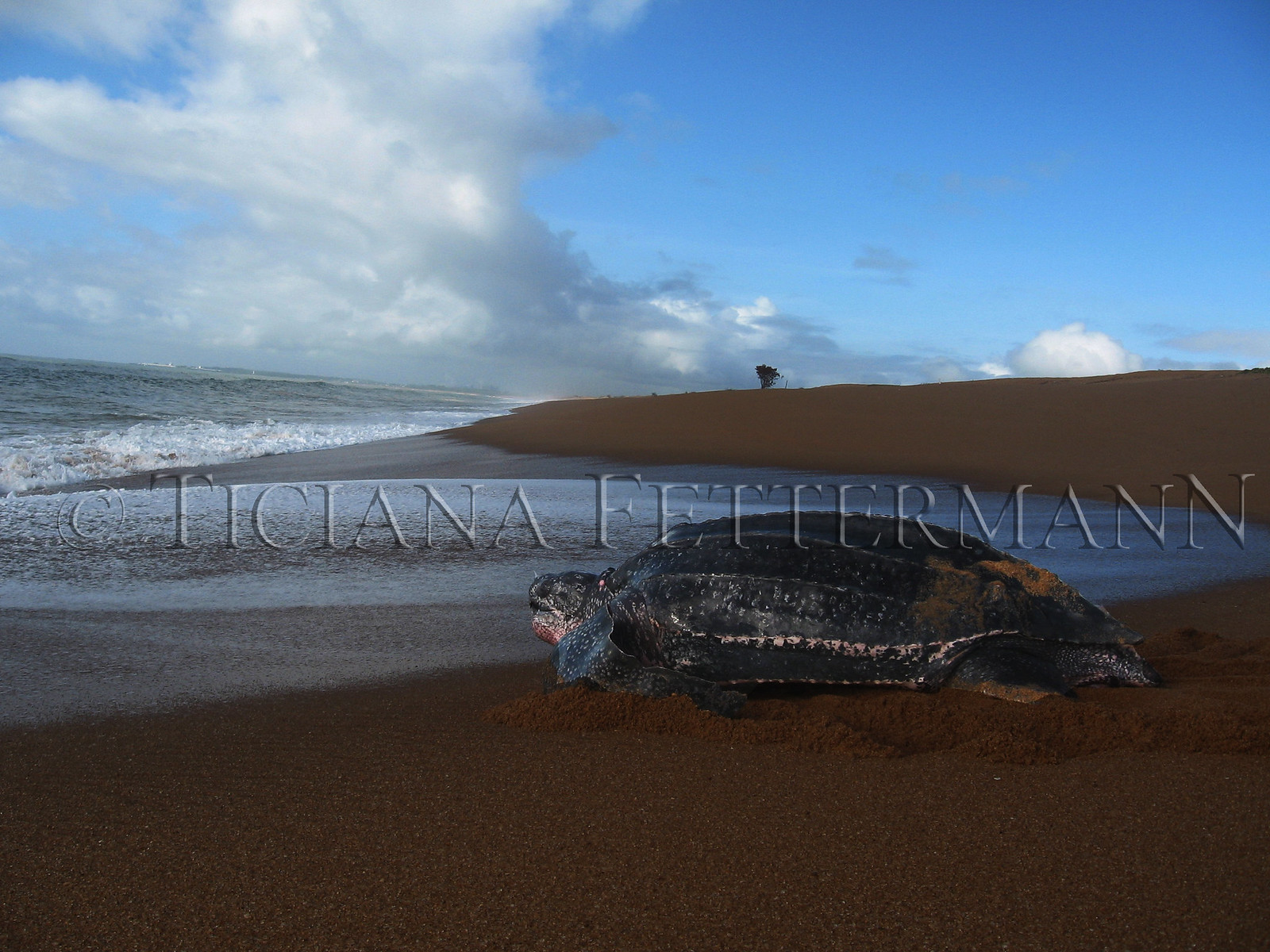A visually striking image depicts a large sea turtle at the verge of entering the ocean, photographed from a ground-level perspective as if the camera were placed on the dark brown sand itself. The turtle, predominantly black with orange spots on its back and a touch of red under its chin, has left distinct flipper tracks behind. The scene is set against a backdrop of rolling waves, under a clear blue sky dotted with scattered white clouds particularly to the left side. In the distance, the sand rises into a hill topped with a solitary tree. Further off, a boat can be seen on the horizon. The beach and water are both strikingly dark in color, with the waves adding a dynamic element to the scene. A copyright message overlays the center of the photograph, attributing the image to Tishana Fetterman.